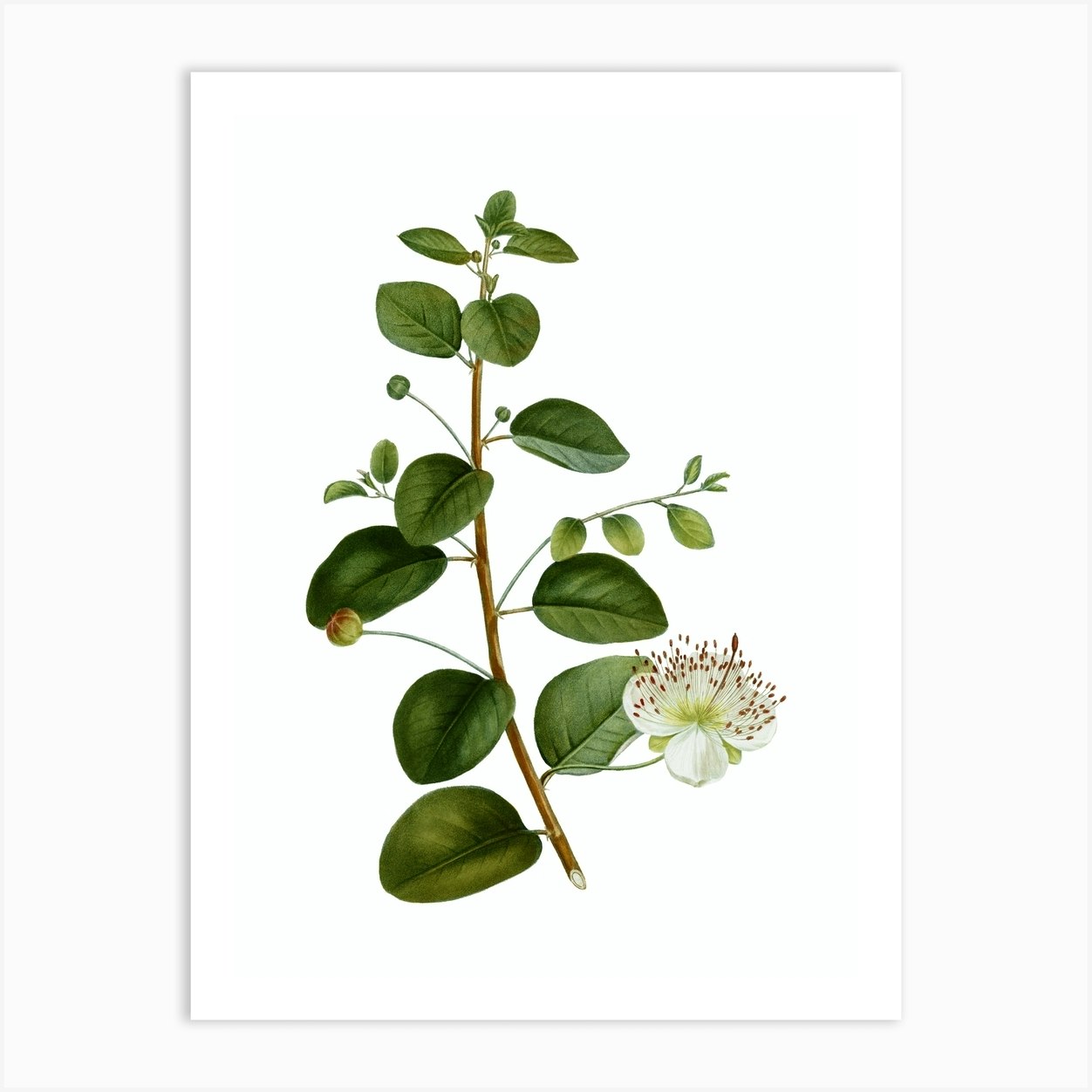The image features a highly detailed, realistic botanical illustration of a dogwood plant. Presented on an off-white, tall rectangular background with a clean white cardstock overlay, the illustration meticulously depicts a single, cut-off branch of the dogwood. The main twig, predominantly brown, extends upward with several smaller branches and an array of green, oval-shaped leaves. Scattered among the foliage are several green buds. A prominent feature of the drawing is one open white flower on the lower right side, showcasing four or five petals and distinct red-dotted stamens at the center. The precise and lifelike rendering emphasizes the unique shape and delicate details of the dogwood plant against the minimalist white backdrop.